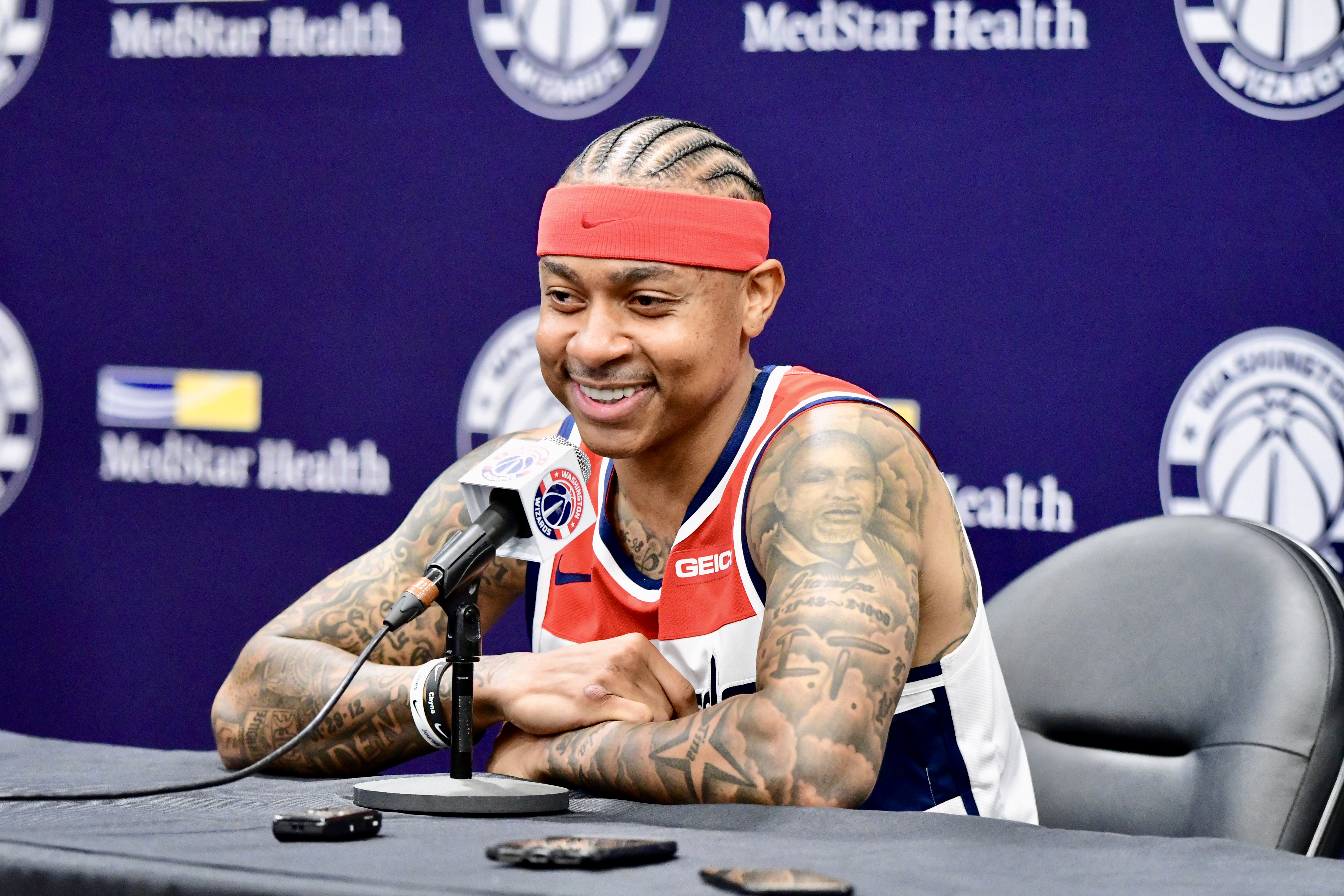In the image, a smiling Black basketball player with cornrows is seated at a gray table, engaging in a press conference. He is wearing a thick red Nike headband, a red, white, and blue tank top with "Geico" on it, and a plethora of tattoos adorning both his arms and chest. Positioned in a gray leather office chair, he is angled slightly from left to right, addressing the media through a black microphone mounted on a stand on the table. The backdrop features a purple wall with multiple advertisements, predominantly displaying "MedStar Health" repeatedly, interspersed with blue and yellow accents and white text. His surroundings include a few items on the table, reinforcing the professional setting, likely connected to either a pre-game or post-game interview session.